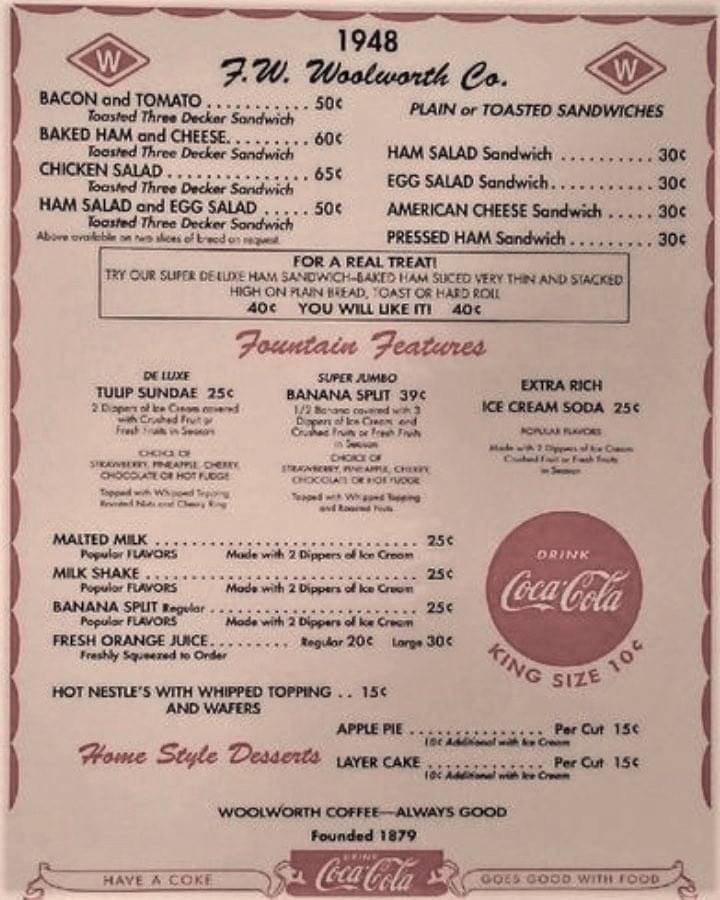Close-up of a vintage, off-white menu with a pinkish hue. The menu, possibly altered by a filter, features a red-bordered edge and displays black and red text. At the top, it reads "1948 T.W. Woolworth, Colorado" in bold black lettering. Various items are listed, with key dishes such as a "Bacon and Tomato Toasted Three-Decker Sandwich" priced at 50 cents and a "Baked Ham and Cheese Sandwich" priced at 60 cents, available plain or toasted. 

In the center, "Fountain Features" is elegantly written in red cursive, highlighting treats like sundaes and banana splits. The affordability of the items implies the menu's historical nature. At the bottom right corner, a prominent red circle labeled "Drink Coca-Cola" in white lettering is visible, with "King-Size 10 cents" beneath it in red. The bottom left corner features "Home-Style Desserts" in red script. Stretching across the bottom is a banner proclaiming "Have a Coke," with "Coca-Cola" in red in the center, flanked by the phrase "Goes Good with Food" on the right.